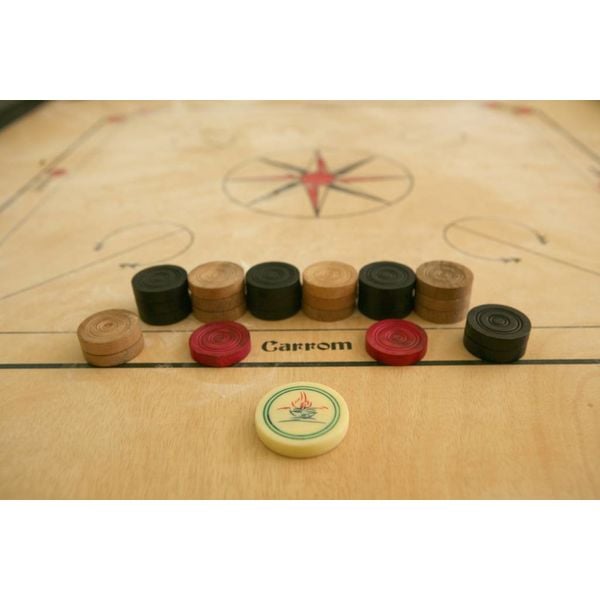The image depicts a wooden Carrom board game in a setting that resembles someone’s home, ready for play. At the center of the board, there is a prominent arrangement of round game pieces. The bottom-most piece is a distinct light yellow color with a green border and features a green and red design. This piece appears to be the main striker for the game. Above this piece, the word "KAROM" is displayed in black letters across a horizontal black line, flanked by two red discs. 

To the left of the word "KAROM" is a stack of two tan tokens, and to the right, a stack of two black tokens. In the background, the board features a large circle with a star motif, comprising red and black arms radiating from the center. Additionally, there is an arrangement of game pieces that form a row along the top of the image; this sequence consists of alternating stacks of black and wooden-colored tokens. The overall setup hints at an imminent game of Carrom, with the board prominently showing a well-organized array of pieces ready for the first flick.